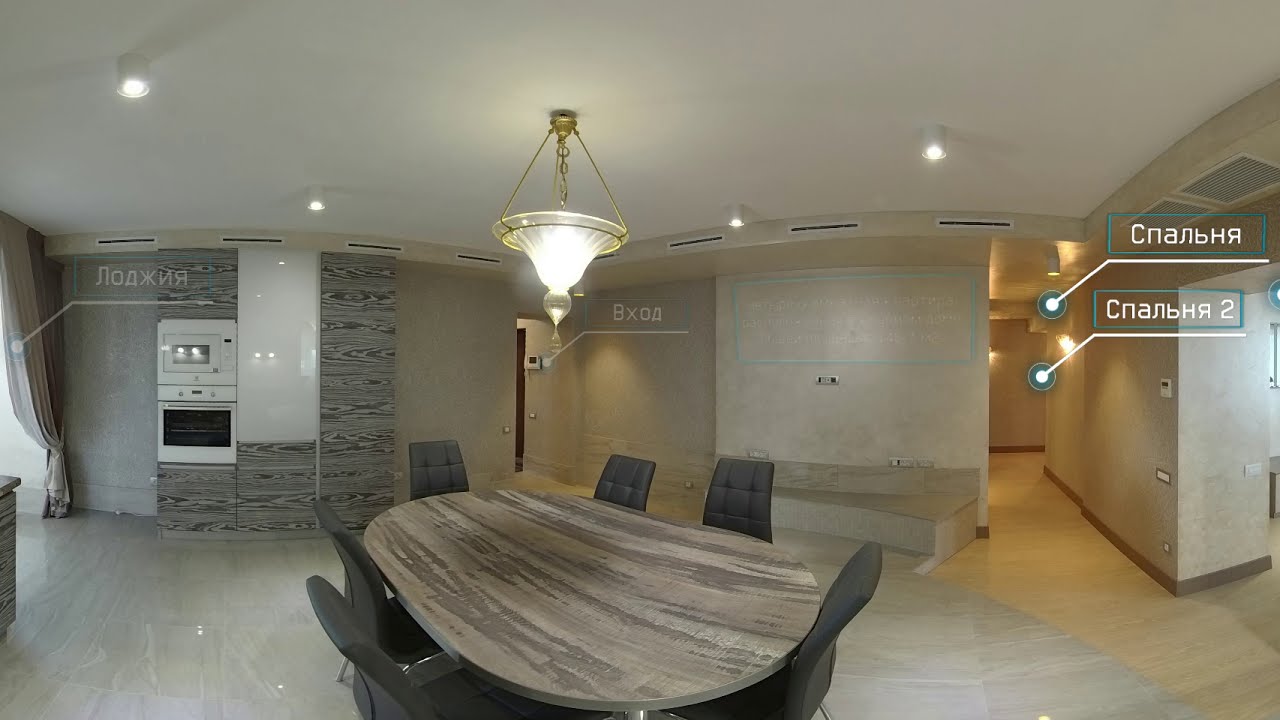This is a horizontal rectangular image showcasing the interior of a modern, stylish apartment room, likely captured with a wide-angle lens. Central to the composition is a large, round table that appears slightly oblong due to lens distortion, surrounded by six grey chairs. The table is positioned near the bottom center, slightly offset to the left. Above the table hangs a simple yet elegant white and gold chandelier.

The color palette of the room is dominated by beige and gray hues, giving it a sophisticated and neutral aesthetic. The light brown table contrasts with the grey chairs, while the floor is a lighter gray, and the walls feature darker gray wood paneling. 

On the left side of the image, an oven is built into the wall, appearing in white, and next to it, light brown curtains suggest the presence of a window just outside the frame. The right side of the image reveals a hallway with what seems to be lockers or cupboards, adding to the functional design of the space. 

Two labels with a white line pointing to specific elements are visible within the room, accompanied by non-English text, possibly Russian, hinting at the room's context—maybe an advertisement or a real estate listing highlighting the apartment's features. The overall scene is well-lit, clean, orderly, and devoid of personal belongings, indicating it might be staged for a property showing.